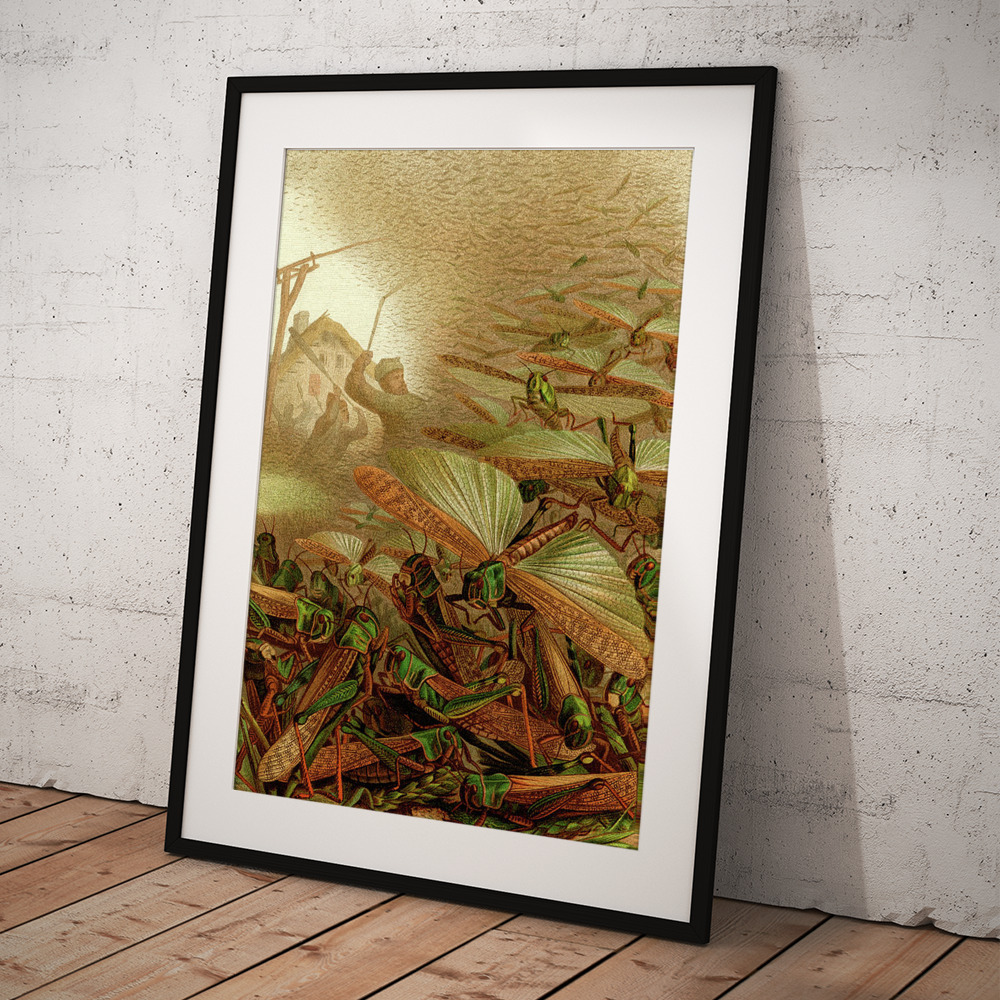The photo depicts a vertical rectangular digital print in a black frame with white matting, leaning up against a scuffed gray wall over a floor made of light-colored wooden planks. The artwork itself is a vivid scene showcasing a multitude of locusts swarming the area, their green heads and brown bodies with light-colored wings prominently displayed. In the upper left-hand corner of the print, three men engage in a futile battle against the locust invasion. One man wields a whip, another brandishes a paddle, and a third holds up a rifle. Behind them, a tan-colored house with a sturdy chimney stands as a backdrop, emphasizing the overwhelming scale of the locust swarm descending from the sky. The dramatic scene captures the chaos and desperation as the men struggle to fend off the relentless wave of locusts.